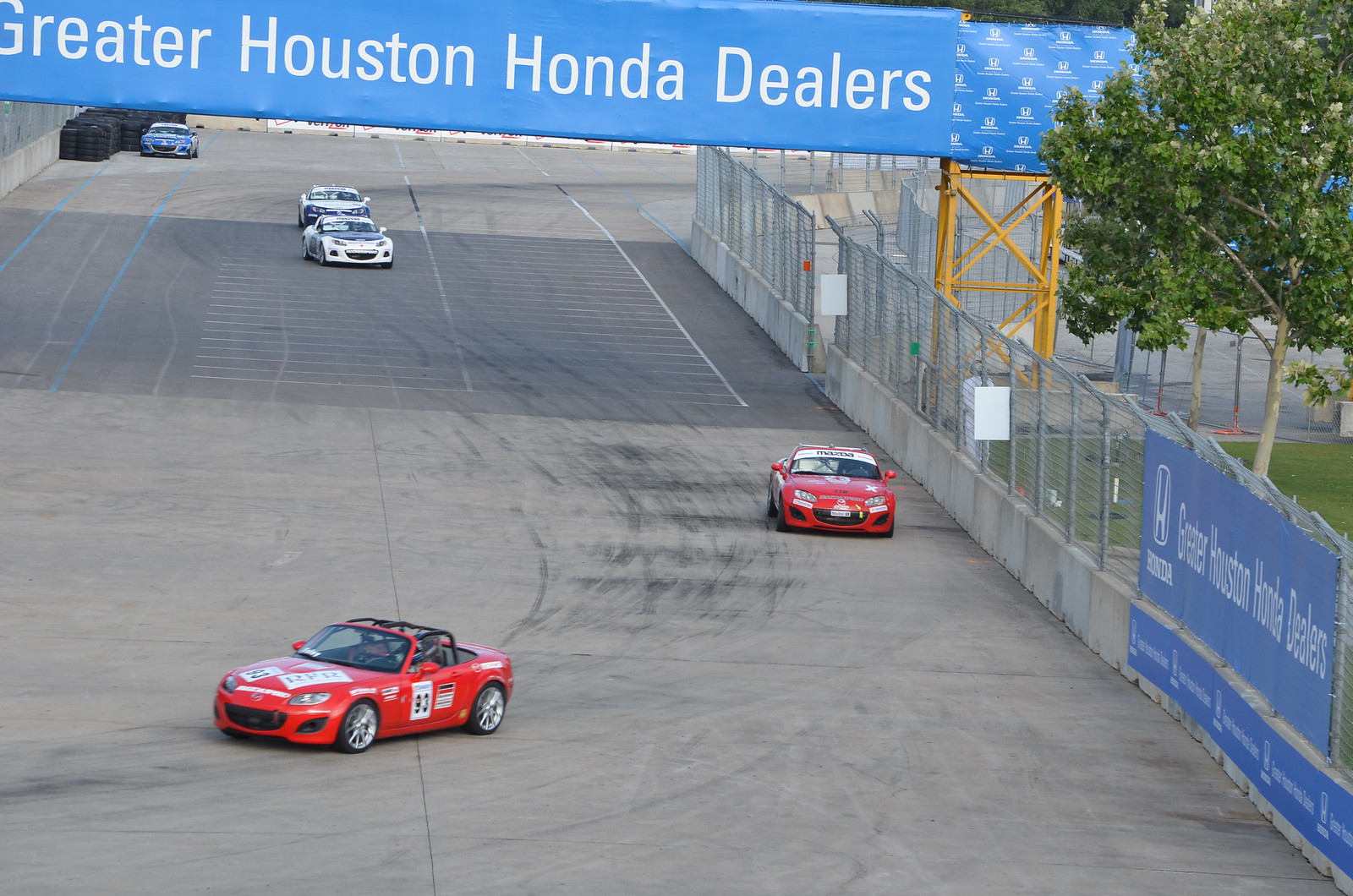This photograph captures an exciting moment on a racetrack featuring several race cars under a vivid blue sky. Spanning across the top of the image, a light blue banner prominently displays "Greater Houston Honda Dealers" in white lettering. Below the banner lies the expansive light gray asphalt of the racetrack, marked with black tire streaks from previous high-speed maneuvers. 

Five cars are visible in the scene: a blue car situated in the back left corner, two white cars positioned one behind the other in the middle, and two red cars—one at the far right and the other near the front left corner of the track. The prominently leading car, a red one, is marked with the number 93 in a white box with black numerals, distinguishing itself as an open-top vehicle with pronounced black roll bars.

The right-hand side of the photograph is bordered by a protective concrete barrier topped with a fence, which also features an additional advertisement for Greater Houston. In the backdrop, a large green tree and a grassy area add a touch of natural beauty to the high-octane scene.